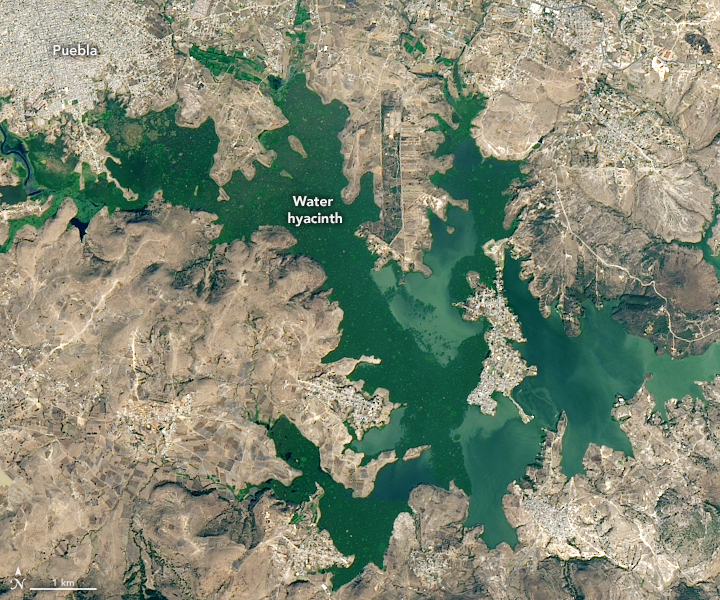A detailed satellite image showcases a geographical area with a mixture of green and gray hues, featuring a prominent body of water labeled "Water Hyacinth." In the upper left corner, the word "Puebla" is clearly spelled out, indicating a possible city or region. The landscape reveals several notable details: numerous roads crisscross the area like veins, groups of houses are interspersed throughout, and extensive stretches of terrain appear eroded. The water body itself is irregularly shaped, with finger-like inlets and a distinct green color, contrasting with the surrounding shades of tan and brown landmasses.